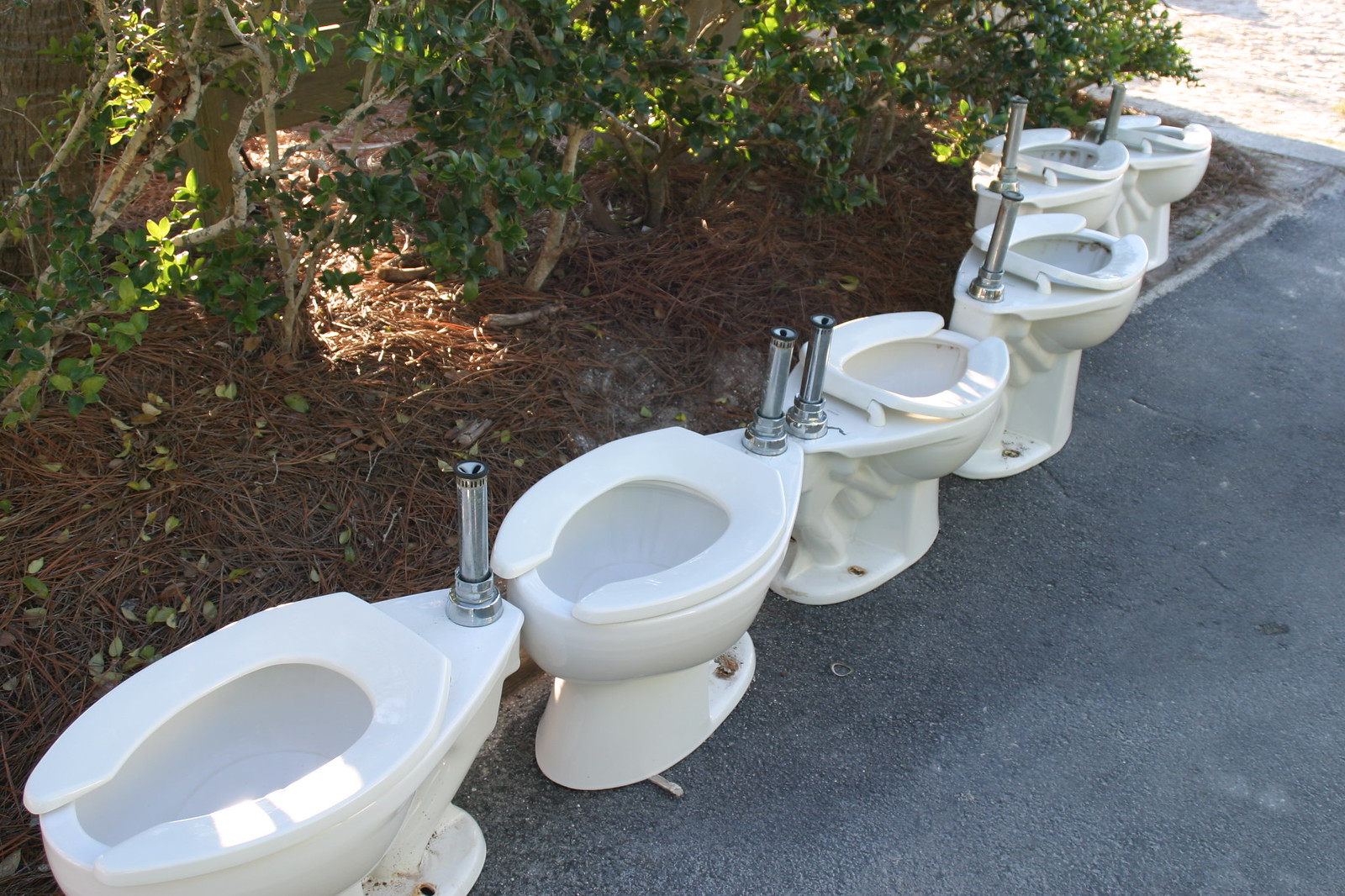This image is a horizontally oriented, outdoor color photograph capturing a row of six used, commercial-style toilets without their top tanks. The toilets are aligned in a diagonal line starting from the bottom left-hand corner and extending towards the upper right corner of the photograph. They are positioned on a dark gray pavement, possibly a sidewalk or the edge of a parking area. Adjacent to the toilets, on the left side, is a garden area with a combination of straw brush, twigs, leaves, and some green shrubs or weeds. The white porcelain toilets feature long, oval seats with a chrome pipe sticking up from the back. Sunlight highlights parts of the toilets, adding contrast to the overall scene. There is no text or additional markings in the image, giving it a potential abstract or modern art quality. The foreground is slightly darker, while the upper right corner of the image is lighter, enhancing the composition.